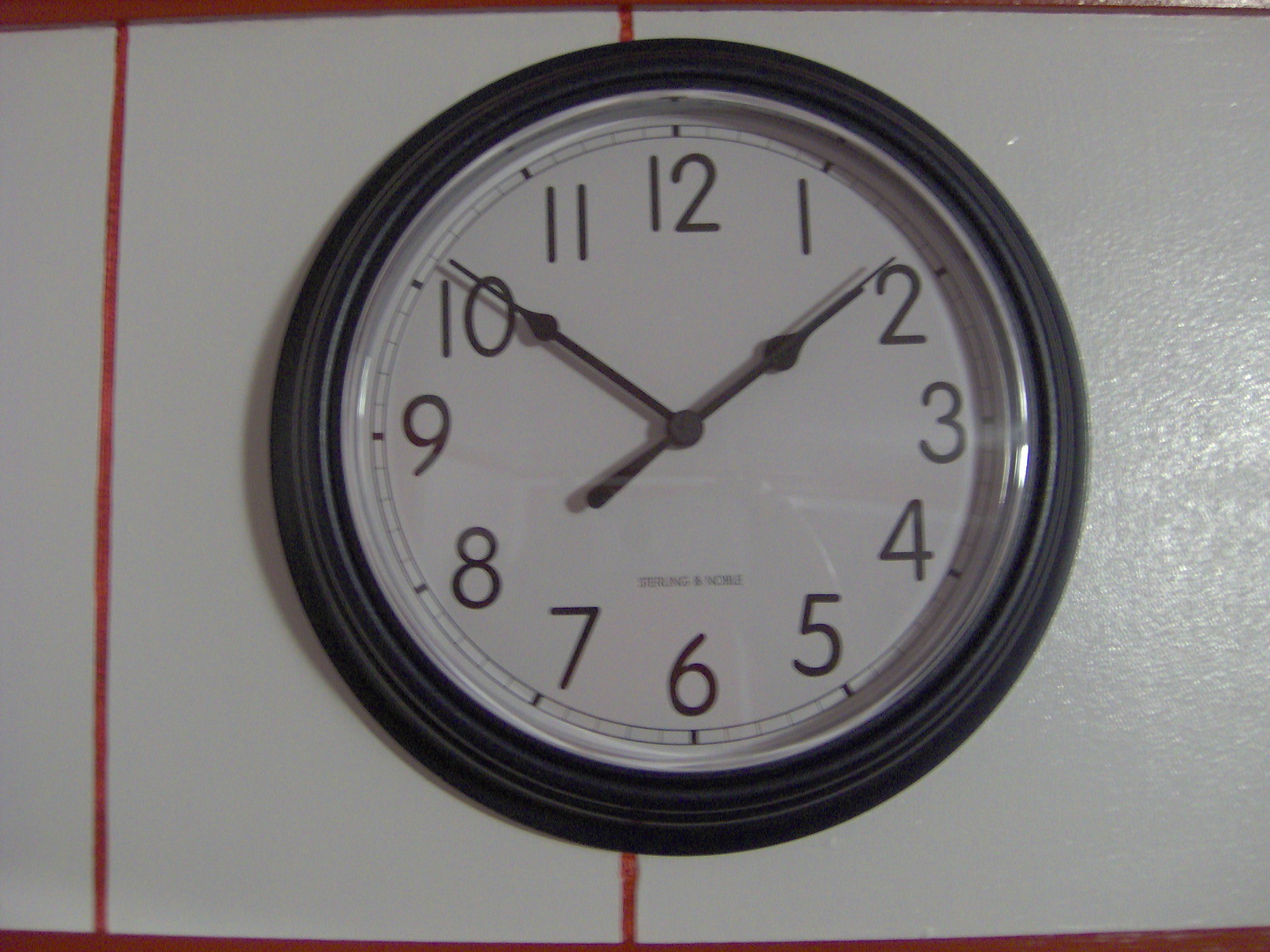The photograph features a prominently displayed analog clock on a wall, which occupies the majority of the image. The wall is tiled in white with an orange-red grout, giving it a textured appearance. The clock, bearing the label "Sterling and Noble," has a black beveled frame encasing a white face. The clock's hands and numerals (ranging from 1 to 12) are in black, with small dash marks indicating each minute and thicker dashes for the hours. It also has a secondary circle indicating the exact minute positions. The larger hand is pointing between 10 and 11, the smaller hand at the 2, marking the time as 1:51, with the second hand just past the 2, around 8 seconds in. The clock is covered with a reflective surface, possibly glass or plastic, which adds a bit of glare to the overall appearance.